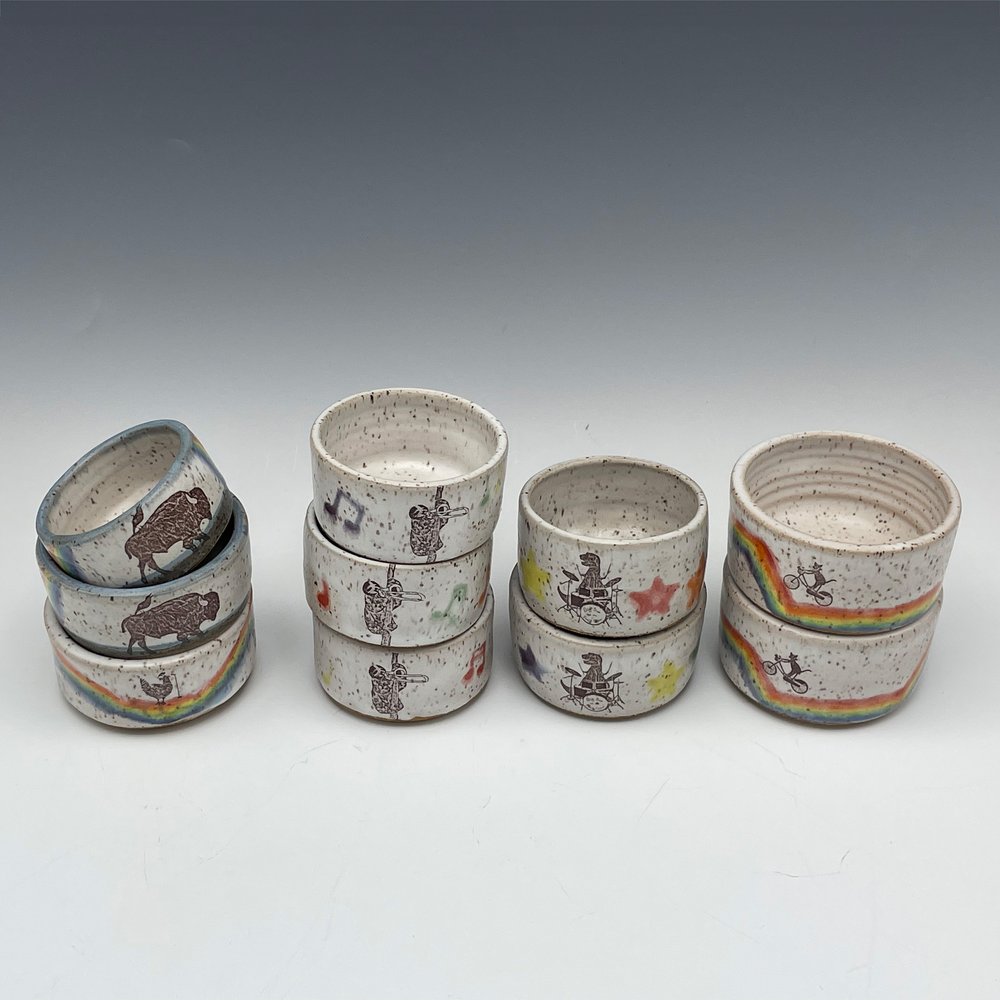The image showcases a professionally photographed arrangement of four stacks of hand-painted ceramic bowls on a light gray to near-white gradient surface, set against a background that transitions from dark to light gray. The bowls are uniform in size and feature a consistent white base with black speckles, giving them a distinctive, cohesive appearance. On the leftmost stack of three bowls, two showcase a blue-rimmed design with images of brown bison, while the bottom bowl features a colorful wavy rainbow with a chicken at its nadir. The adjacent stack of three bowls displays musical notes and a sloth playing a trombone, adding a whimsical touch. The third stack contains two bowls adorned with various colored stars, featuring illustrations of a T-Rex playing drums. The final stack of two bowls depicts a cat riding a bicycle atop a rainbow. Each bowl's unique, detailed design highlights its handmade and hand-painted craftsmanship.